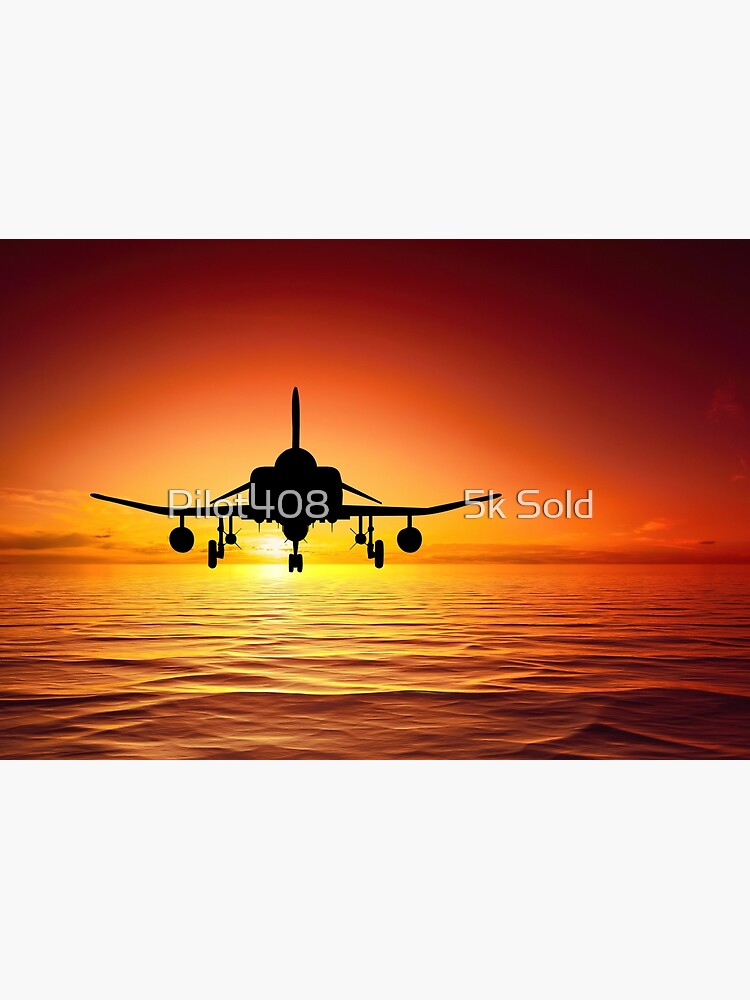The image depicts a striking silhouette of a U.S. F-4 Phantom fighter plane, a rare aircraft from the 1960s, captured in mid-landing with its gear down. The plane, viewed from the rear, is detailed with dihedral wingtips and outfitted with storage tanks and missiles across its wings and main airframe. The horizon behind the aircraft signifies an open body of water, devoid of any land. A vivid sunset saturates the sky in gradients of yellow, orange, and red that deepen into dark red at the edges. The calm water surface reflects this warm palette, with subtle ripples evident. The scene is overlaid with various X and plus sign watermarks, enhancing the layered composition. Overall, the silhouette of the F-4 Phantom dominates the scene, standing starkly against the vibrant backdrop of the setting sun.